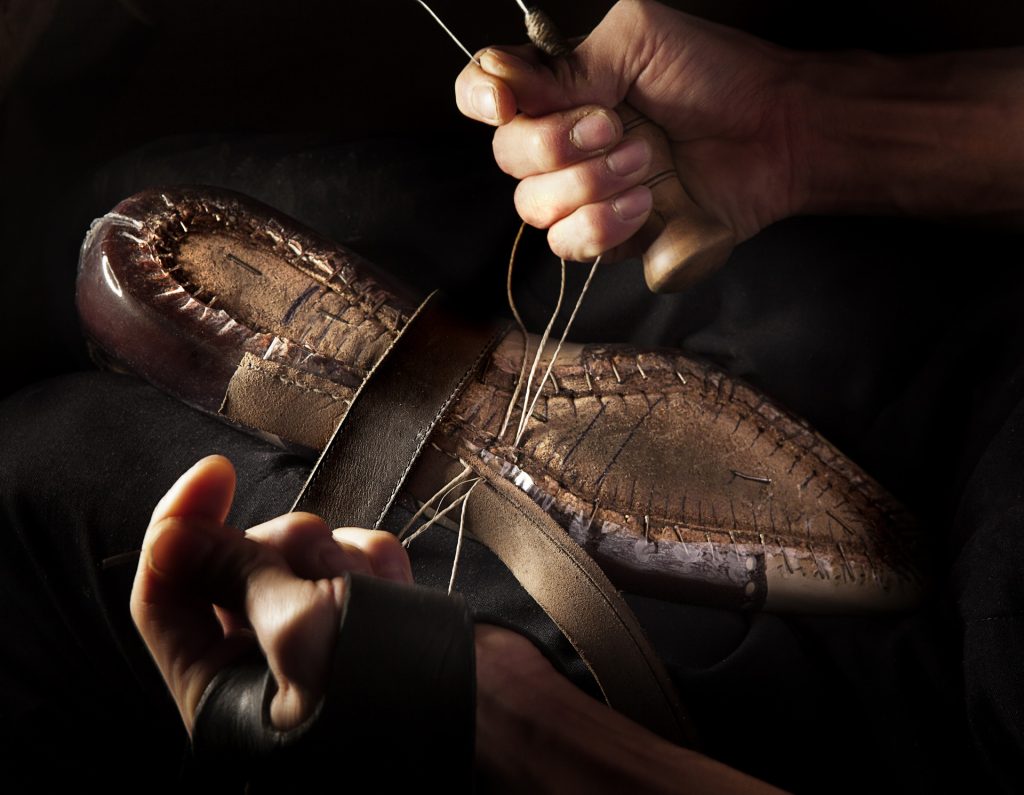This professionally taken photograph captures an intricate close-up of a cobbler’s skilled hands at work. The image focuses on a man's hands, with his left hand wrapped in a brown leather strap and his right hand holding a wooden-handled tool. The cobbler is meticulously stitching the underside of a well-worn, brown leather shoe, which is positioned upside down with the sole facing the camera. The black background, illuminated by a spotlight, accentuates the beige and tannish pink tones of the worker's hands and the rich hues of the leather. The shoe’s sole has been partially removed as the cobbler threads leather strips back into place, repairing the shoe with careful precision. The reddish-brown heel of the shoe catches a slight glint, adding to the detailed and textured appearance of the handmade shoe.